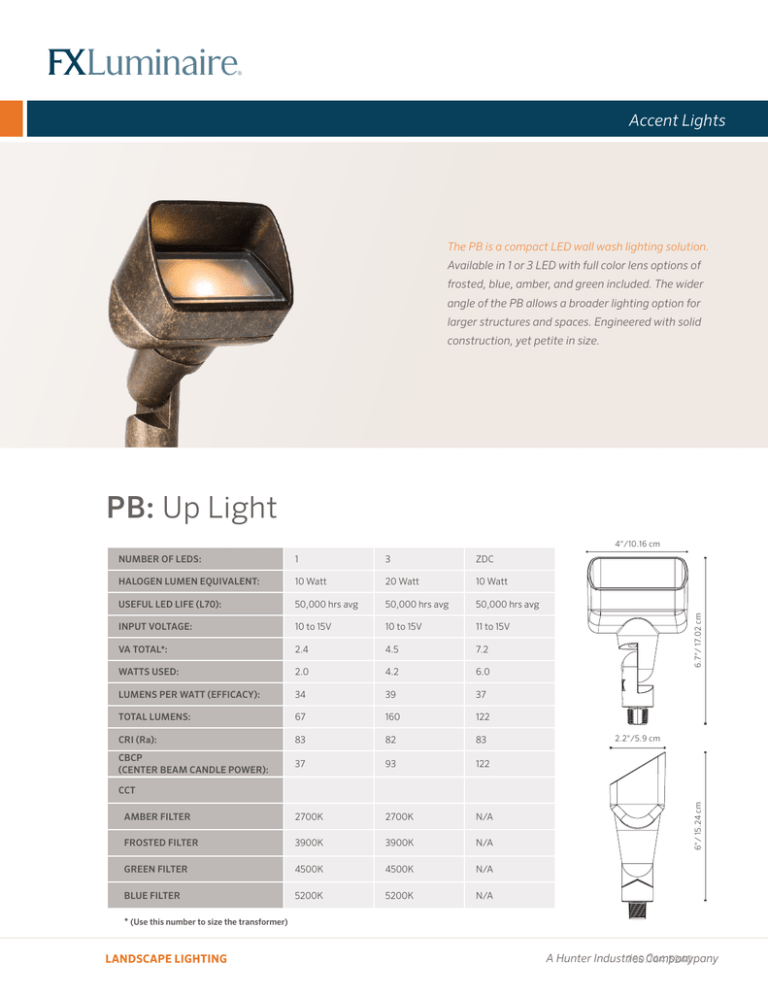The image features a promotional piece for FX Luminaire, prominently displayed against a stark white background. In the top left corner, "FX Luminaire" is written in bold, dark blue text. Below this, an accent strip runs horizontally, starting with a gradient of orange fading into white, and transitioning into a deep blue that spans the rest of the strip. On the right side of this strip, the words "Accent Lights" are elegantly presented in white font.

Beneath this strip lies a beige rectangle showcasing a product. On the left side of this rectangle, a compact LED wall wash light is prominently illuminated. Adjacent to the light, the text describes the PB as a versatile and compact LED wall wash light solution, available with options for one or three LEDs. The product offers a variety of full-color lens options, including frosted blue, amber, and green. Its wider angle is ideal for covering large structures and spaces, and it boasts a solid yet petite construction.

Further details on the beige rectangle highlight the technical specifications:
- **Product:** PB Uplight
- **Number of LEDs:** 1, 3, and ZDC
- **Halogen Lumine Equivalent:** 10 watts, 20 watts, and 10 watts respectively
- **Useful LED Life (L70):** 50,000 hours on average
- **Input Voltage:** 10 to 15 volts and 11 to 15 volts

This detailed caption enhances the understanding of FX Luminaire’s PB Uplight, emphasizing its design, versatility, and technical specifications for prospective users.